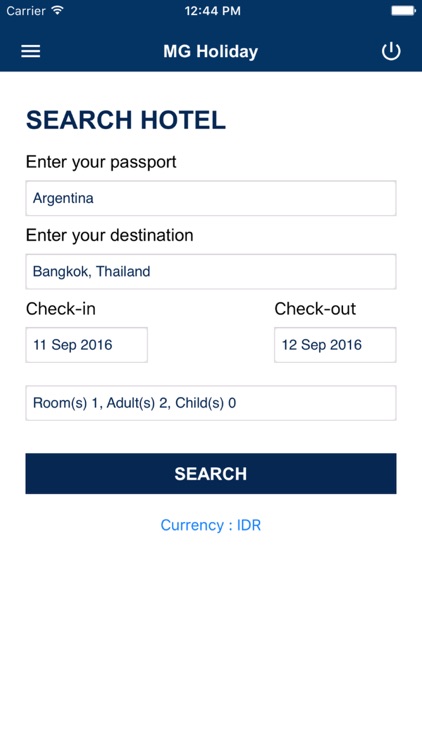At the very top of the image, there is a long dark blue rectangle. In the upper left corner of this rectangle, the word "Carrier" is displayed. Centrally located within this dark blue bar is the time, shown as "12:44 PM." To the far right side, there is a nearly full battery icon with a white symbol inside it. 

Below this, the image is centered around uppercase letters "MG," with the word "Holiday" beside it. Directly underneath, in bold navy blue uppercase letters, the phrase "SEARCH HOTEL" is prominently featured. Beneath this, in black text, the prompt "Enter Your Passport" is written. An open rectangular area follows, inside which the word "Argentina" is featured in blue text.

Subsequently, the phrase "Enter Your Destination" is displayed, followed by another rectangular box with blue text reading "Bangkok, Thailand." On the left side, there is a label for "Check-In," with the date "11 September 2016" displayed below it. To the right of this, "Check-Out" is labeled with the date "12 September 2016."

The next rectangle contains information regarding the room: it specifies "Room(s)" followed by "Adults: 2, Child: 0." Beneath this input area is a long dark blue search bar with the word "SEARCH" in white text at its center. Below the search bar, in light blue text, the label "Currency" is followed by two dots and the abbreviation "IDR."